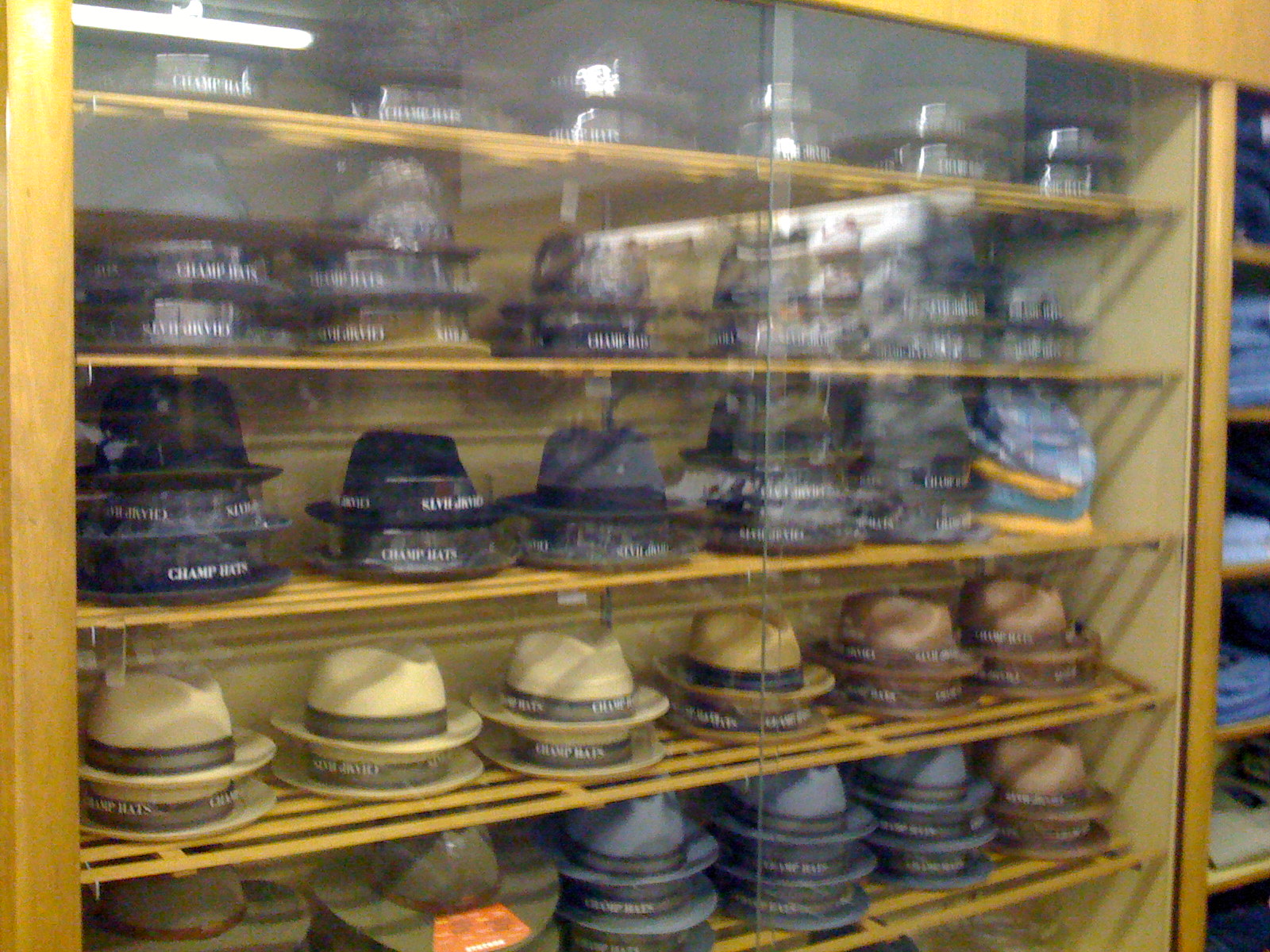The image features a wide display of neatly arranged hats within a glass case that has a brown border and shelves made from slotted wood. The cabinet, positioned against a wall, contains five rows of hats, meticulously organized by color and style. The hats, predominantly fedora and safari styles, vary in hue from dark blacks and tans to vibrant blues and browns, some with decorative bands and leather strips, while others are plain or labeled. The different rows highlight specific color schemes: the bottom shelves predominantly feature blue and brown hats, while the second row includes tan and brown varieties. The top shelves, though slightly obscured by a reflection that reveals an outdoor scene with trees and sky, consist of darker shades. A notable detail is an olive green hat with an orange paper and white writing on it, positioned at the front. Additionally, there is a partial view of another section on the right, showing shelves possibly containing pants, not enclosed by glass. The overall effect combines the captivating interior display with the subtle interplay of outdoor reflections.